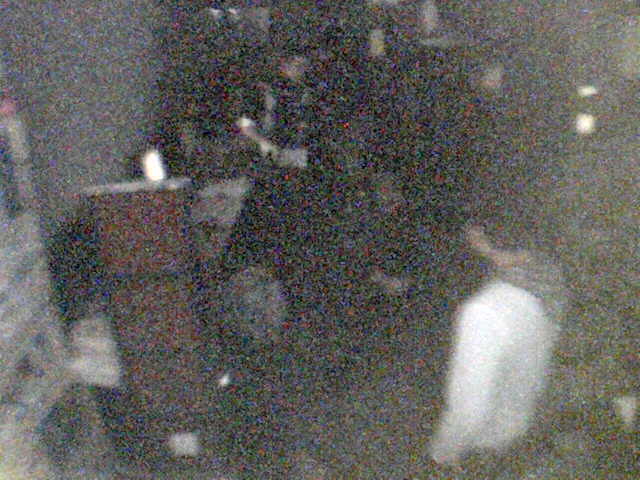In this extremely grainy and blurry photo, we can discern a few details despite the overall difficulty in making out the scene. In the bottom right-hand corner, there is a person with brown hair wearing a white shirt. This person appears to be facing away from the camera, with their arm at their side, and they might be wearing a black scarf around their neck. There seems to be another person toward the center of the photo, partially visible with a black shirt, and an arm noticeable amid the blurriness. The setting could potentially be a get-together or gathering, suggested by the faint outlines of additional people whose heads and forms are vaguely discernible. On the left side of the image, there's a noticeable tall orange object with a silver top, which is hard to identify precisely due to the graininess. There's also mention of what could be three stacked boxes or crates, possibly forming an organizer or podium-like structure. The backdrop includes gray walls and what looks like a long table against the wall. Light is coming from the top right, potentially from two square light sources or a lamp, casting white specks of light amidst the predominantly dark and shadowy scene.